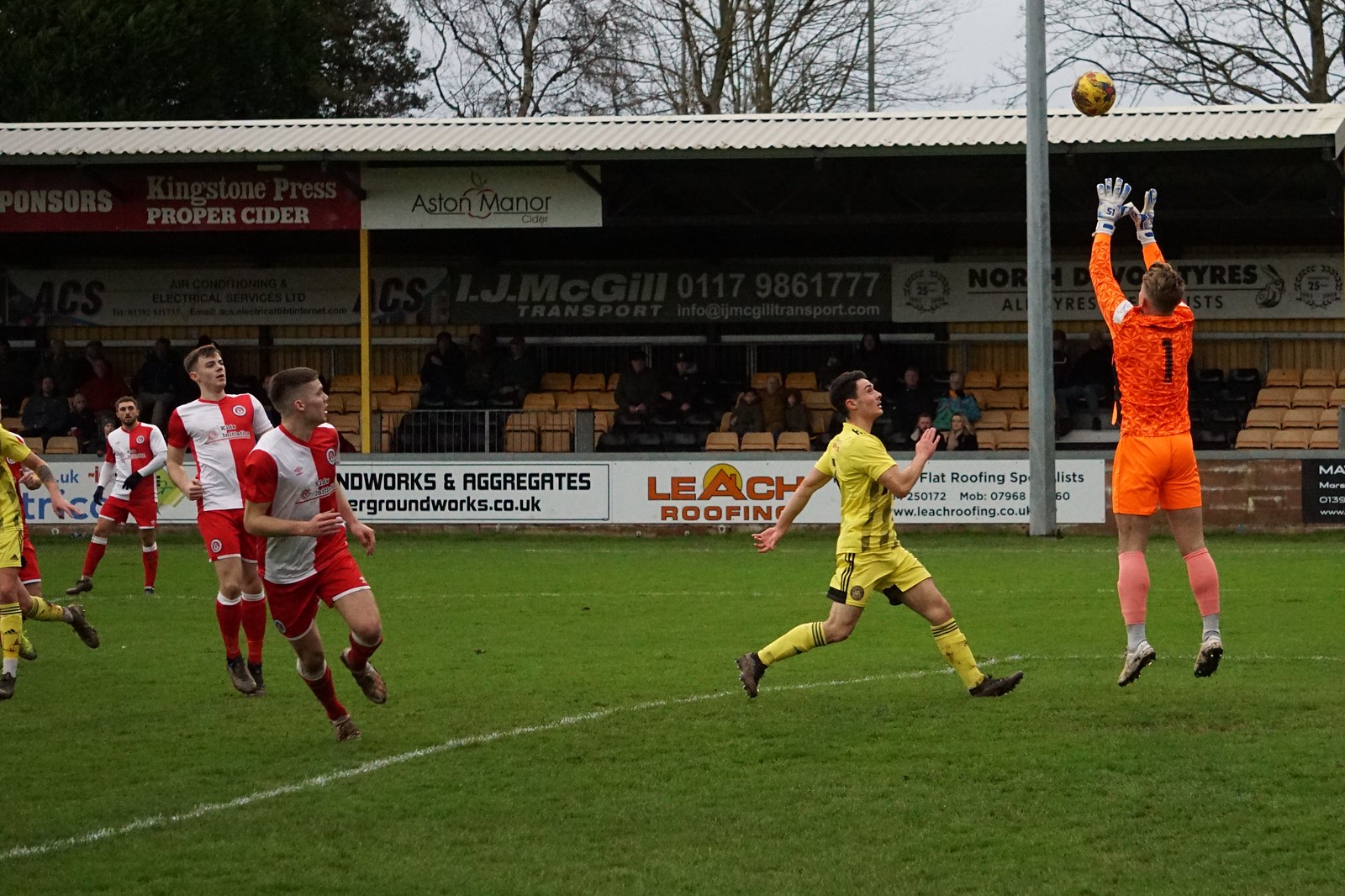In this dynamic photograph of a soccer game, the central focus is on the goalie in an orange jersey, marked as number one, leaping into the air with both hands extended, attempting to catch a mid-air soccer ball. The ball, tinted yellow, hovers just above the goalie. To the goalie's left, a player in a yellow and black uniform is sprinting toward the action, while several players in white and red jerseys are also fixated on the ball, running backwards to position themselves defensively. The game unfolds on a verdant green field marked with crisp white lines. In the background, a modest stadium with only four rows of seats is sparsely populated, about one-third full. Behind the stands is a short advertising wall featuring sponsors such as Leach Roofing, Kingston Press Proper Cider, Ashton Manor Cider, and I.J. McGill Transport, with some advertisements partially obscured by the players. Above the seating area, a covered roof offers shelter to the spectators, contributing to the intimate, close-knit atmosphere of the venue.